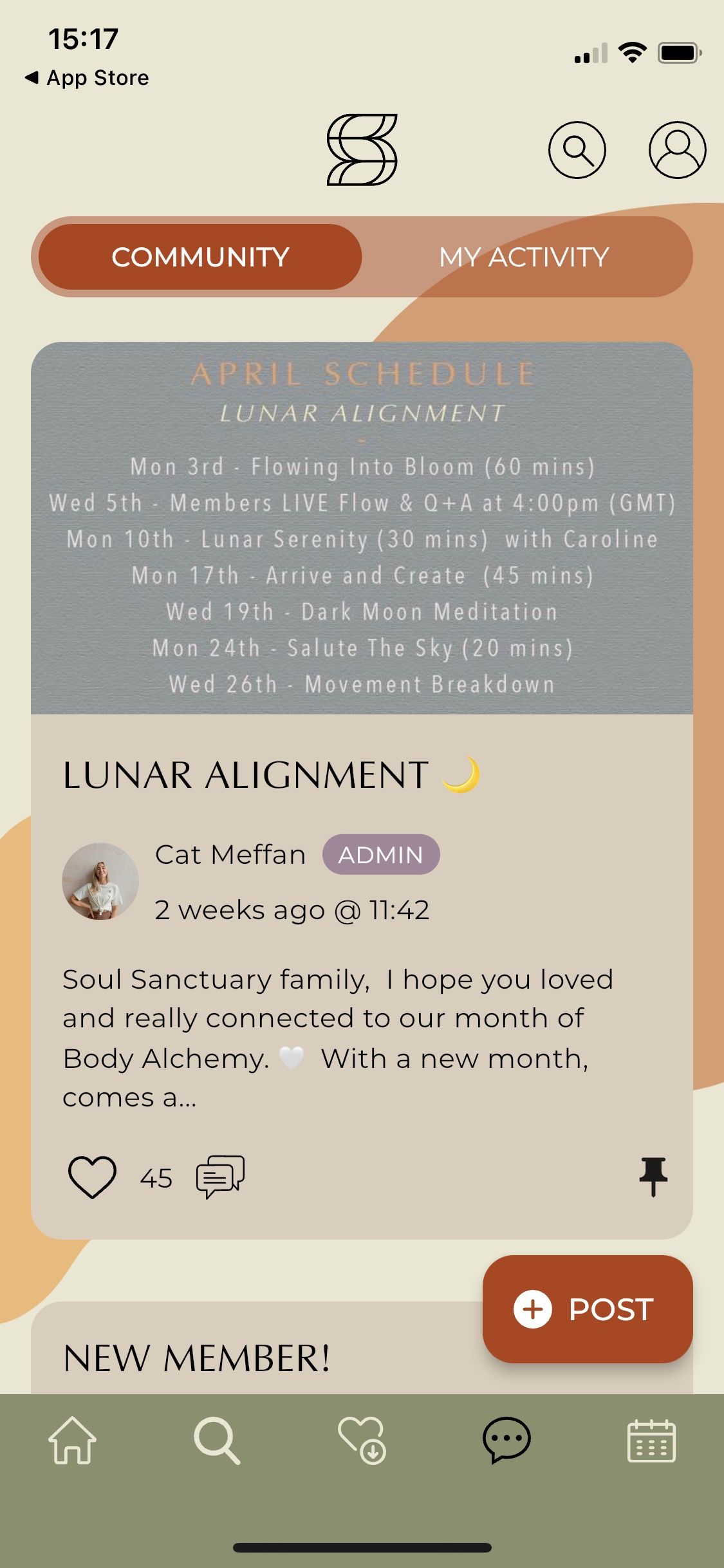A mobile device screen display showcases a vibrant background featuring a blend of beige, light brown, and a light olive green shade. In the upper left corner, the time reads "1517," indicating 3:17 p.m. Just below the profile icon, a rectangular button with curved corners stands out, colored in a rich brown hue. The button has white text, with "Community" written on the left and "My Activity" on the right. Underneath this button, there is a window also designed with curved corners. The top half of the window is gray, presenting white text, while the bottom half transitions to a light shade of beige, displaying black text.